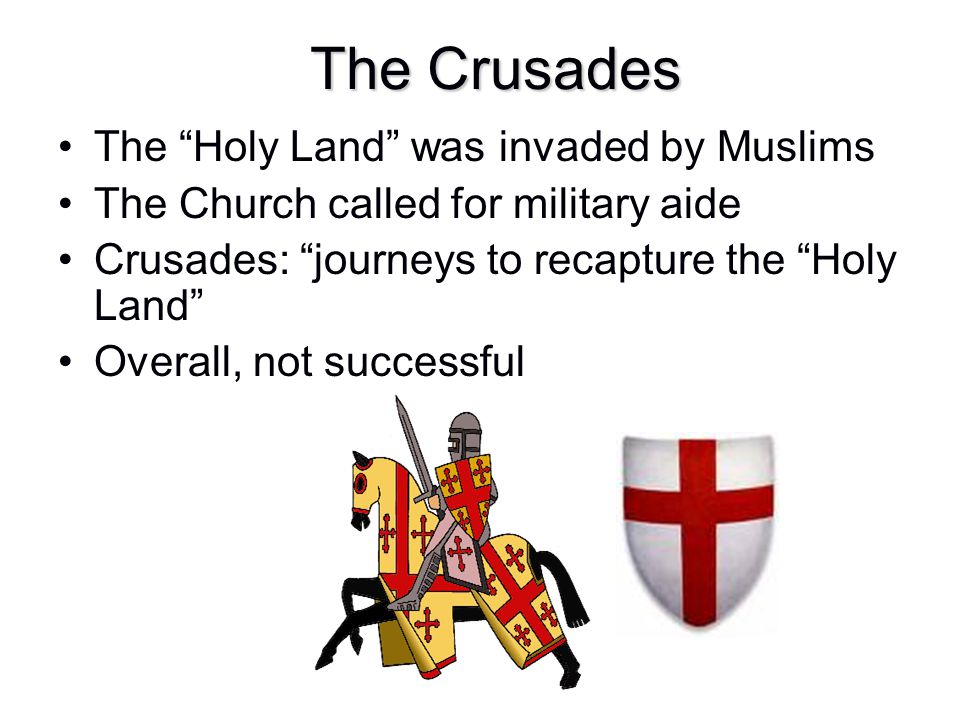The image appears to be a PowerPoint slide designed for a classroom setting, featuring a detailed overview of the Crusades. The background is plain white, providing a clean and uncluttered look. At the top center, the slide prominently displays the title "The Crusades" in bold black print. Beneath this title are four bullet points aligned vertically on the left side, each marked by small black circles. These points, written in black text, read as follows:

1. "The Holy Land was invaded by Muslims."
2. "The Church called for military aid."
3. "Crusades: Journeys to recapture the Holy Land."
4. "Overall, not successful."

Below the text, towards the lower section of the slide, are two images. On the left, there is a cartoon depiction of a knight in full armor riding a black horse, which is dressed in a garment featuring red crosses on a yellow background. The knight holds a sword and wears a helmet. To the right of this image is a shield with a white background, adorned by a red cross. The overall arrangement of text and images is well-organized, typical of an educational slide aimed at teaching students about historical events. The color scheme includes black, white, yellow, red, gray, and some orange, enhancing the visual appeal and clarity of the slide.